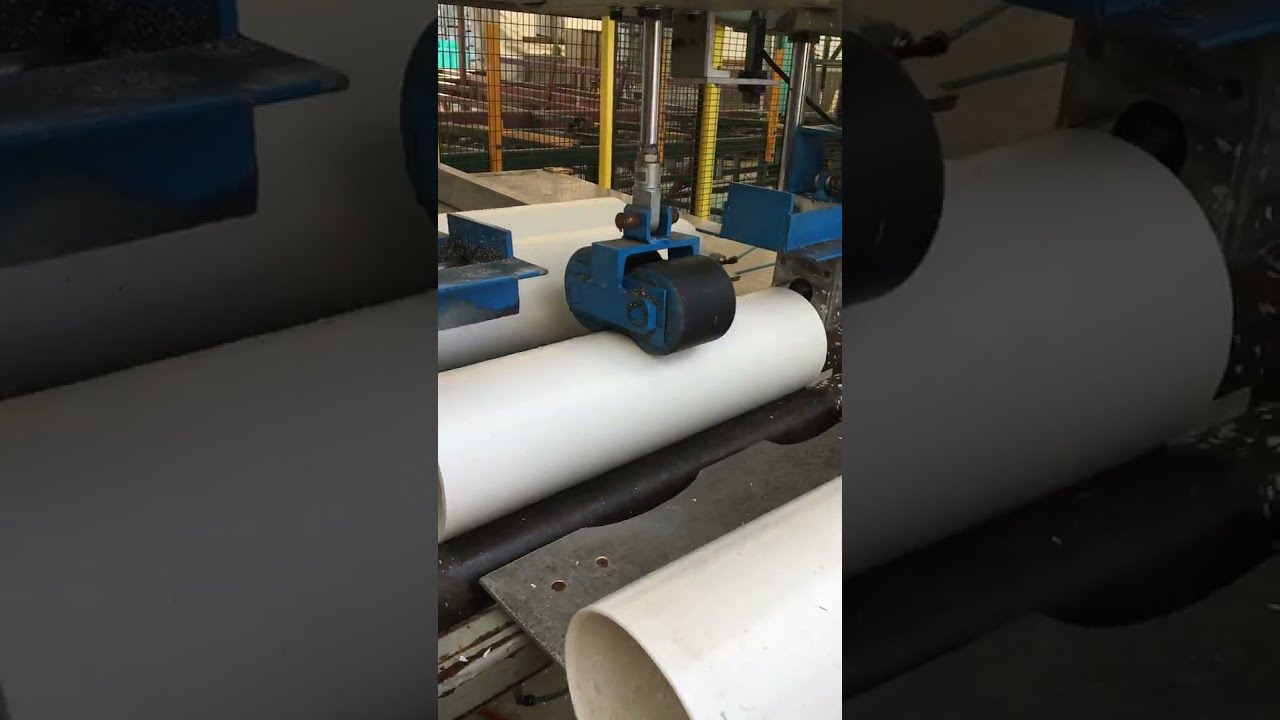The image captures the interior of an expansive industrial warehouse or factory with bright, natural light filtering in. Central to the scene is a notable piece of blue machinery featuring two small black rollers attached above which press down onto larger white cylindrical rollers, each about one foot in diameter. These white rollers, positioned horizontally, rest on additional black rollers beneath them, which are mounted on metal plates. Surrounding the main machine are various other industrial equipment and machinery, some showing signs of wear and rust, indicating prolonged use. The background reveals storage cages and various supplies essential for the industrial processes conducted here. The environment is devoid of people, suggesting that operations may be controlled from a distance or during inactive hours. The entire setting is characterized by a mix of vivid colors including blue, black, white, gray, yellow, green, and orange, contributing to a bustling yet organized industrial scene.